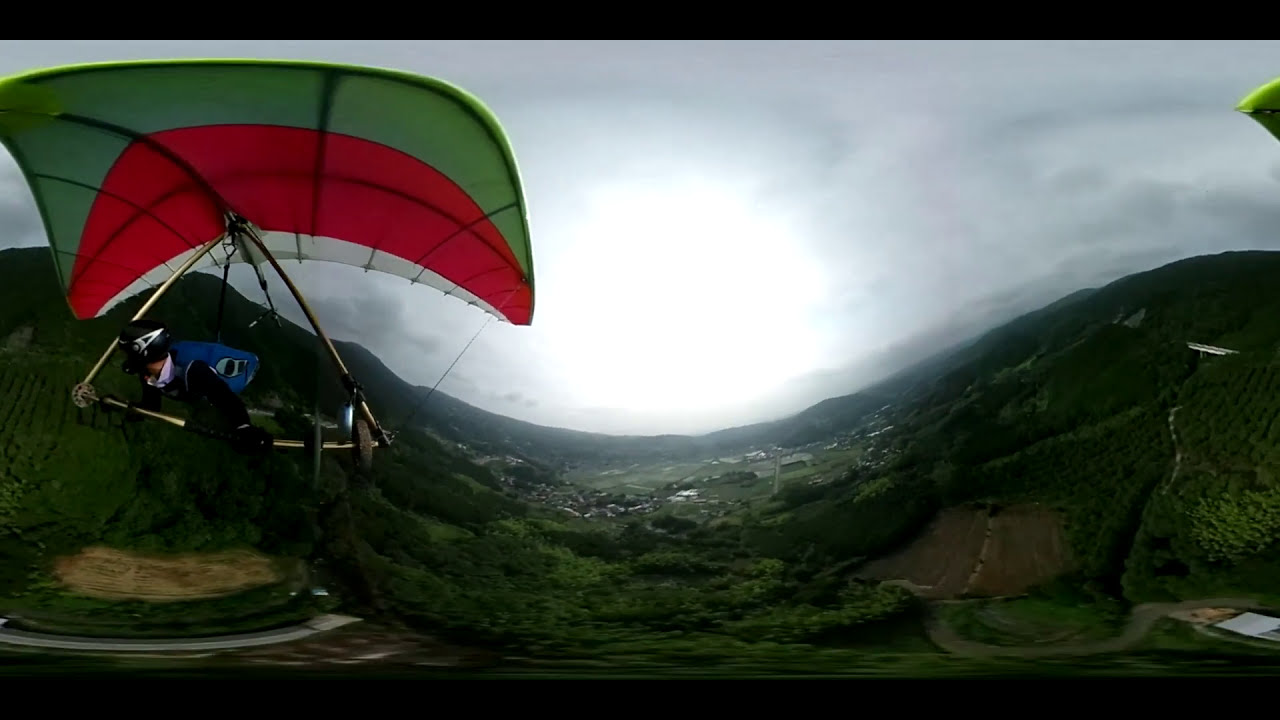This panoramic photo captures a thrilling moment of a person paragliding over a verdant landscape at dawn. The paraglider, dressed in a blue shirt and wearing a helmet, is positioned in the top left corner of the image, gripping the control bars of a green sail adorned with red and white stripes. Below, the scene unfolds with rolling hills blanketed in lush greenery, while a valley stretches out between them. The left and right sides of the picture display grassy hills, and far below, small houses dot the landscape, hinting at distant human habitation. The sky above is overcast with a thick layer of grayish-white clouds, but the sun's rays are beginning to pierce through, casting a gentle light over the scene. Adding to the sense of adventure, another hang glider is glimpsed at the edge of the frame, emphasizing the shared exhilaration of soaring above the tranquil, hilly terrain.